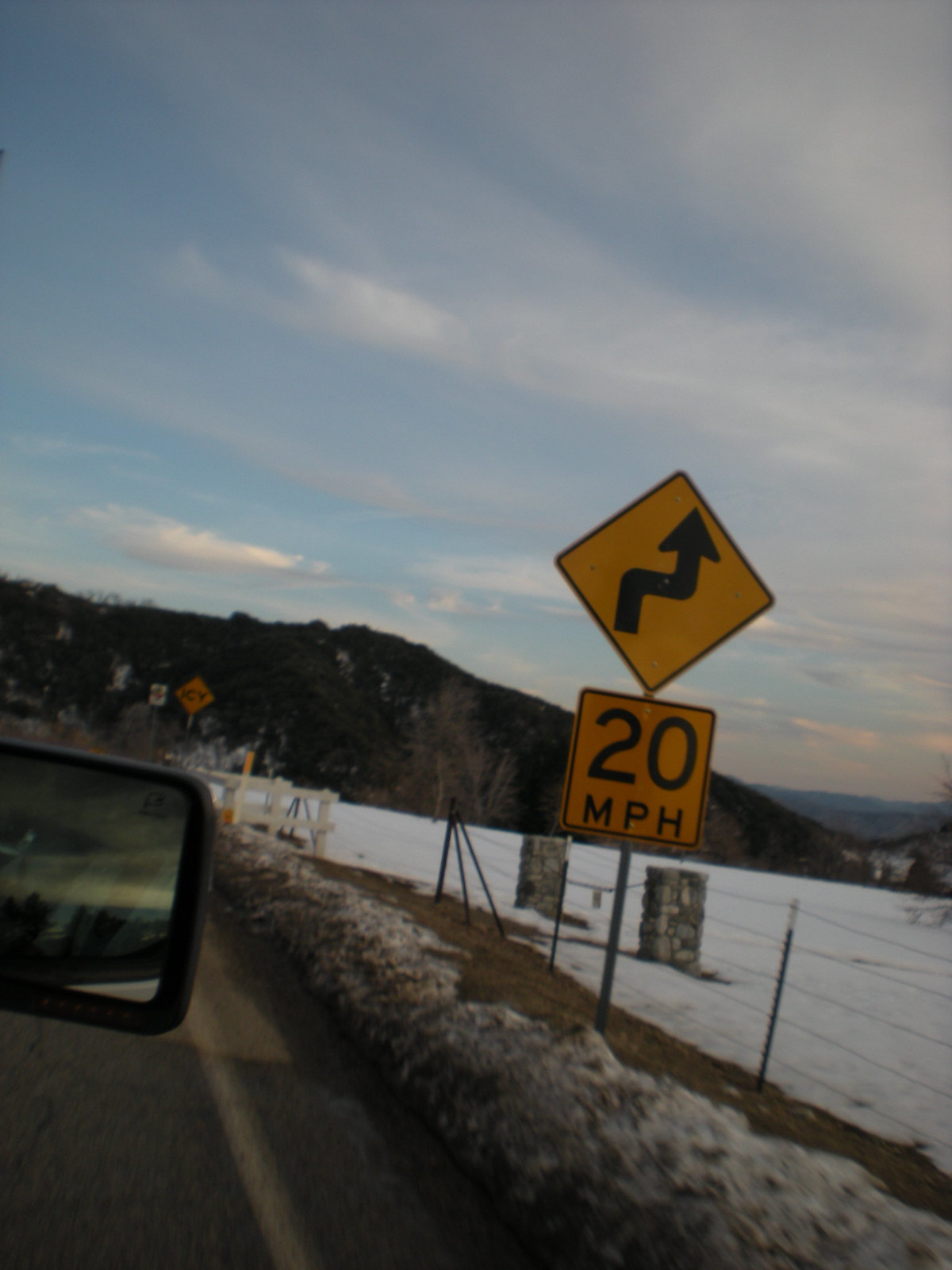In this image, captured from the passenger side of a vehicle, we first notice the rearview mirror with a black, square-shaped outline reflecting the gray road. To the right of the road, a small snowbank is visible, followed by a sign mounted on a gray pole. The sign features a yellow square with "20 MPH" written in black text, and above it, a diamond-shaped sign displays an arrow that points upward, horizontally, and then has a vertical transition capped with a triangle. The right-hand side of the image reveals a snowy landscape with white-covered ground leading up to a small hill or mini-mountain, which appears brown. The sky above transitions from predominantly gray on the right to mostly blue on the left, providing a striking contrast with the wintery scene below.